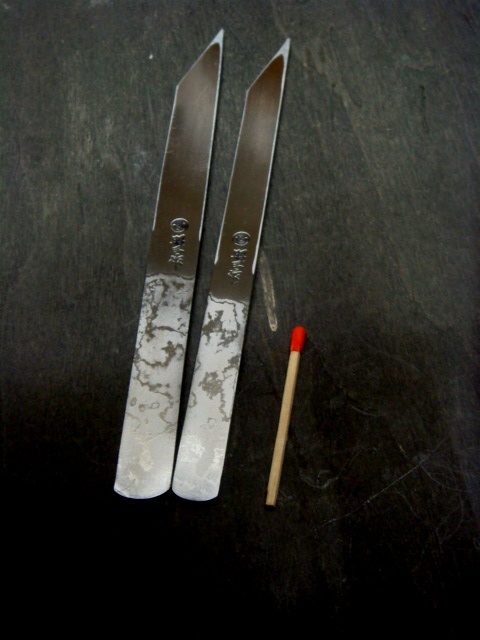The image depicts a black wood table with a slightly scratched but otherwise shiny surface. The wood features strips of varying shades, with some parts lighter and others darker. On this table lie two metallic objects resembling knives or letter openers, each about 3 to 5 inches long. Their handles display a white and gray marble pattern, and the blades, covered in protective plastic, feature a polished metal surface that ends in a sharp point. The blade of the left opener is marginally wider than the right. A matchstick, made of light tan wood with a red tip, lies to their right, providing scale. An embossed oriental logo can be seen on the top part of the metal, above the handle.